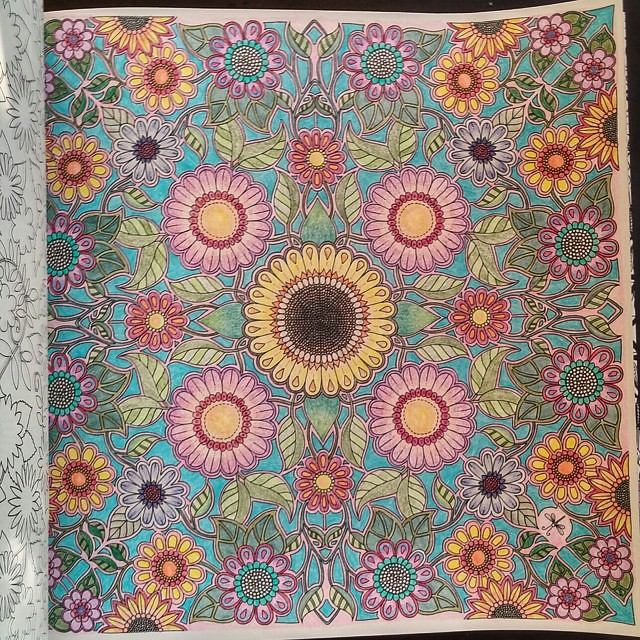The photograph showcases a meticulously colored page, resembling the intricate designs of adult coloring mandalas. The artwork appears to be completed with colored pencils, evident from the subtle shading and vibrant hues. At the heart of the composition is a stylized sunflower, boasting an array of detailed petals and dark spots in the center. Surrounding the sunflower in the four corners of the page are stylized pink daisies. Extending outward are additional smaller daisies, yellow flowers, and an assortment of purple and blue blossoms. The entire piece is intricately connected by intertwining, twisty green leaves. The slightly curled page indicates that it is an actual coloring book page on paper. Even the background is thoughtfully filled in with a soothing teal blue color, completing the detailed and aesthetically pleasing artwork.